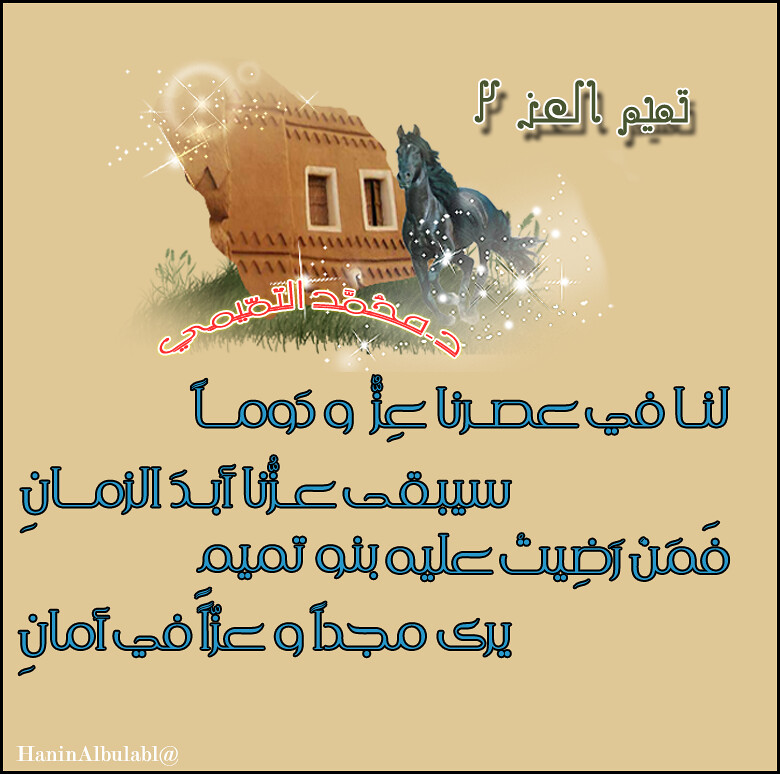This is an image, likely a poster or cartoon-like, featuring a central figure of a black horse with a white star on its forehead, running on grass. The background is a light tan or brown, and the scene includes part of a brown building with white trim around windows that have no glass; one of the windows appears partially opened, constructed with wooden interiors. Sparkling light or sparkles are noticeable around the horse and near the building's front part, suggesting motion or magic. The horse is positioned more on the upper right of the image, surrounded by blue and red text in a foreign language, possibly Arabic. The writing is predominantly blue, with some sections in red and black, and it includes the phrase "Hanan Alulabi." Overall, the picture captures a dynamic and somewhat mystical scene with detailed, colorful elements that evoke a sense of both movement and cultural context.